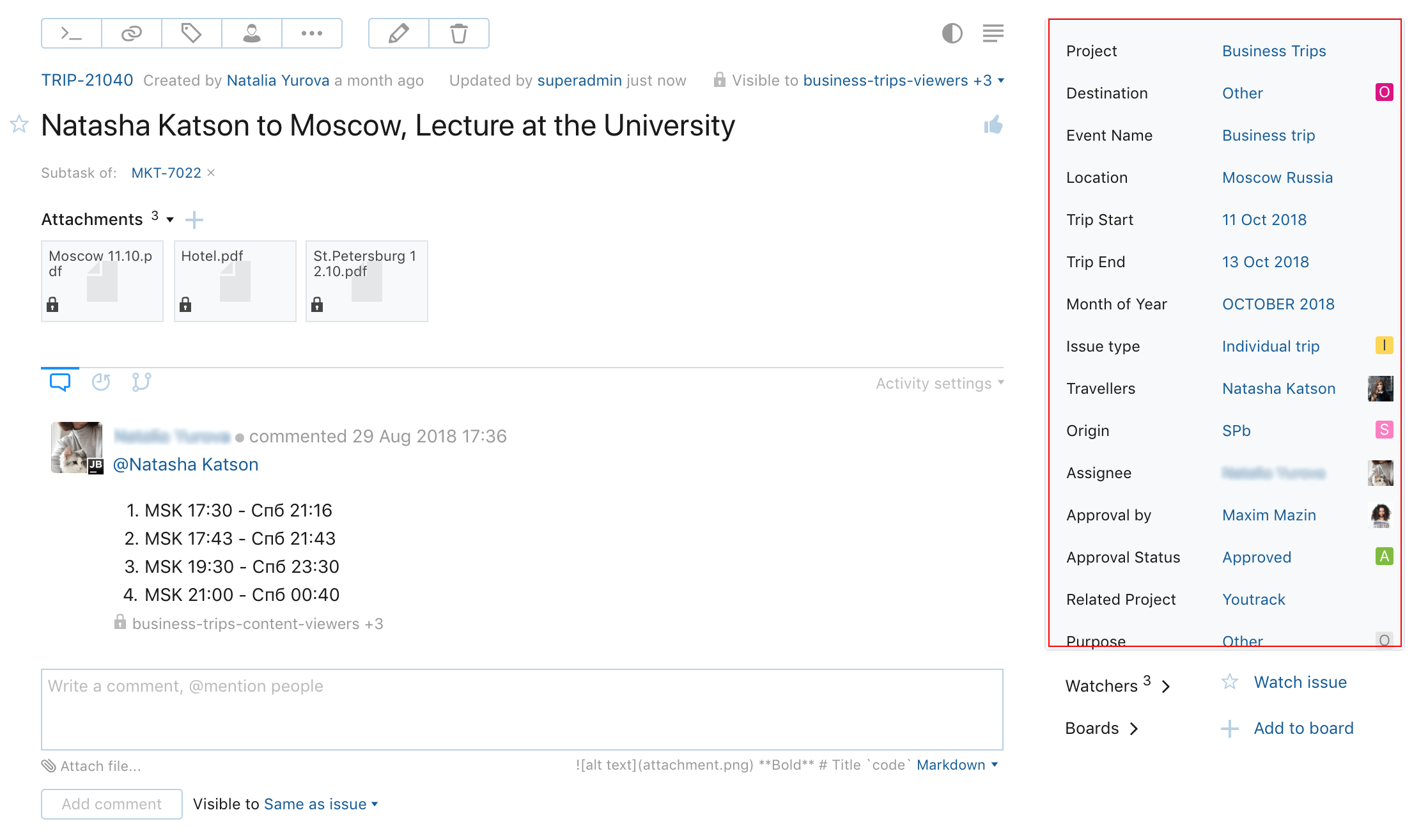The image depicts a project page titled "Subtask of MKT7022." It features text indicating an attachment count of three. This project involves Natasha Katzen and is affiliated with the Moscow Electoral University. Below the main text, several fields are available for writing comments and attaching files. To the right of the image, there are multiple details listed:

- **Projects:** 
  - Business Trips
  - Destination: Other Events

- **Trip Details:**
  - **Name:** Business Trip
  - **Location:** Moscow, Russia
  - **Start Date:** 11th October 2018
  - **Trip Date:** 13th October 2018
  - **Month & Year:** October 2018

- **Approval Details:**
  - **Approved by:** Maxim Mazin
  - **Approval Status:** Approved